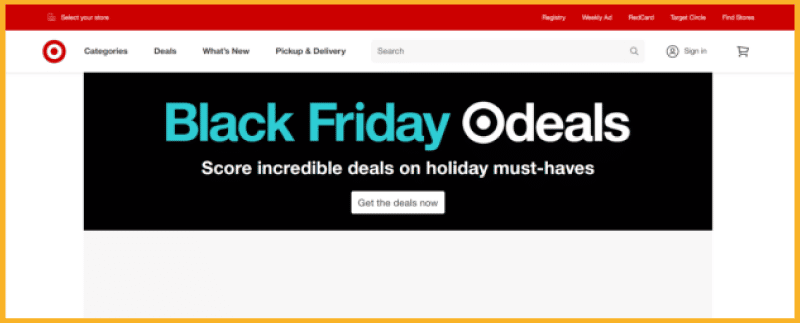A cropped screenshot displays a section of the Target website, highlighting a Black Friday promotional banner. The banner stands out with its black background and contrasting white text, except for the phrase "Black Friday," which is rendered in a light blue font. It features a prominent "Get the deals now" button in white, which has black text. Surrounding the banner, the rest of the website's interface is primarily white. The familiar Target logo is positioned in the top-left corner, accompanied by the site's top navigation bar that includes categories such as "Categories," "Deals," "What's New," "Pickup & Delivery," and a search bar. To the right, there are additional features such as a "Sign In" button and an empty shopping cart icon. Above the main navigation bar, there is a narrow red bar containing several links, though their small size makes them difficult to read in this resolution. Overall, the screenshot captures the essence of Target's website during their Black Friday sales event.